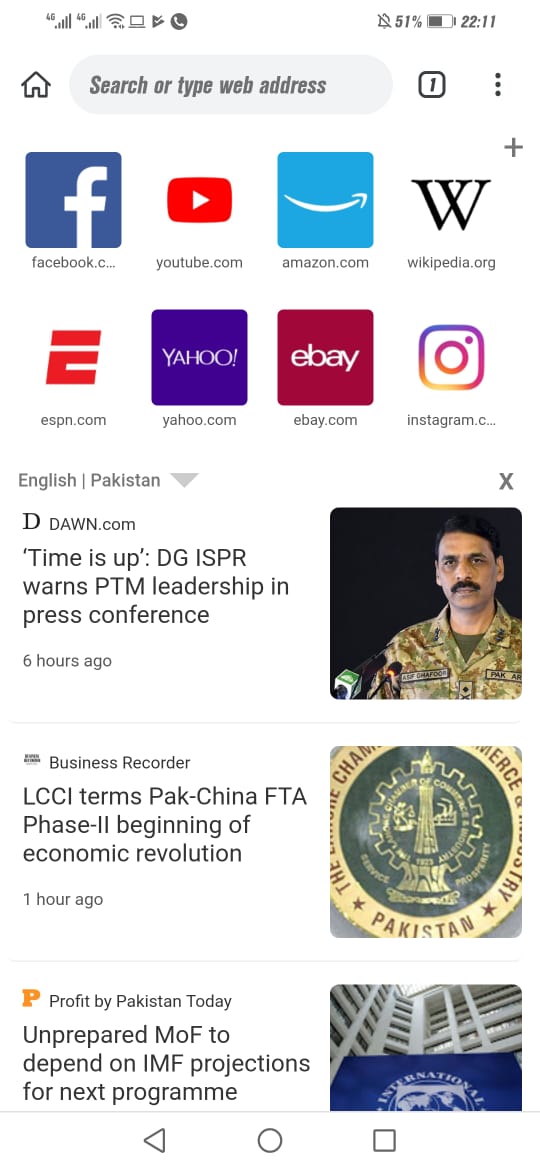This screenshot features a web browser interface. At the very top is the search bar with the prompt "Search or type web address." Below the search bar, there are two rows of website icons. The first row includes icons for Facebook, YouTube, Amazon, and Wikipedia. The second row features icons for ESPN, Yahoo, eBay, and Instagram.

Further down, the screen displays three articles arranged vertically. Each article features a headline on the left and an accompanying image on the right. Above each headline is the source of the article. The first source is "Dawn.com," followed by "Business Recorder," and the third source is "Profit by Pakistan Today."